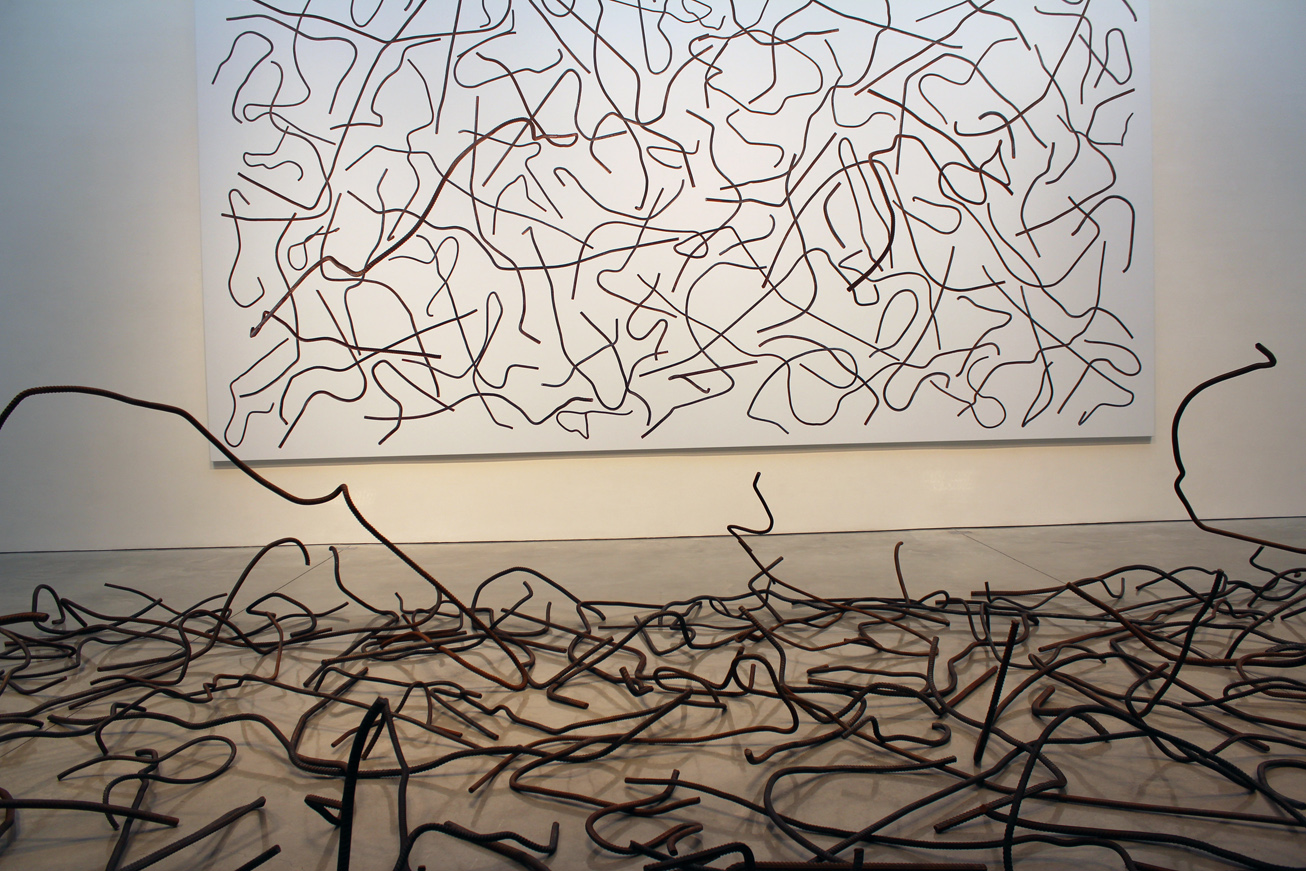This color photograph depicts a modern art exhibit that features a large white canvas mounted on a white or cream-colored wall. The canvas is densely covered with irregular black squiggly lines that lack any discernible shape or pattern, creating a chaotic yet intriguing visual. Mirroring this chaotic design, numerous dark brown or black metal rods, intricately twisted to match the squiggly lines on the canvas, are positioned on the floor in front of the artwork. These metal pieces appear as if the black squiggly lines from the painting have materialized and scattered across the floor, creating a cohesive and immersive artistic installation that blurs the line between two-dimensional and three-dimensional art.